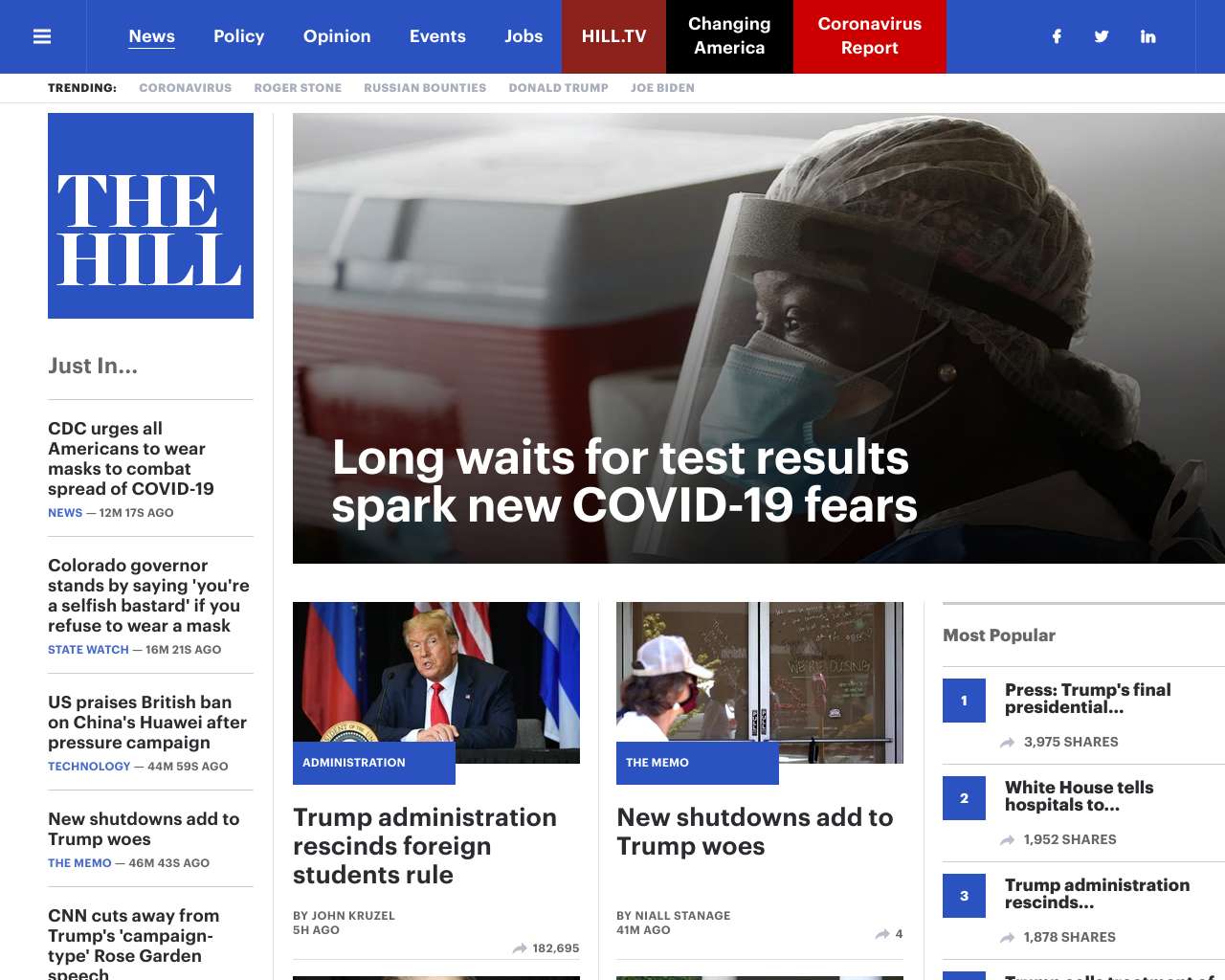This is a detailed screenshot from the web page of a newspaper called The Hill. The page features a blue header at the top with a menu bar that includes the following options: News, Policy, Opinion, Events, and Jobs. Specific sections such as "Hill TV" in a red box, "Changing America" in a black box, and "Coronavirus Report" in a red box are highlighted within the menu.

On the far right of the header, there are icons for Facebook, Twitter, and Instagram. The sidebar on the left side of the page prominently displays The Hill’s logo at the top, followed by a list of four or five articles. The first article in the sidebar reads, "CDC urges all Americans to wear masks to combat spread of COVID-19." The second article, by State Watch, is titled, "Colorado governor stands by saying you're a selfish bastard if you refuse to wear a mask."

The main content in the right pane of the page features a large image of an African American woman wearing a double mask. The accompanying text headline reads, "Long waits for COVID test spark new COVID-19 fears." Below this primary article, there are two additional picture articles. The first one, tagged "Administration," includes a picture of Donald Trump with the title, "Trump Administration rescinds foreign schedule rule," authored by John Kruzel and posted five hours ago. The second article, tagged "The Memo," reads, "The shutdown adds to Trump woes," and is positioned to the right of the first.

Additionally, on the right side of the page, there is a chart listing the most popular articles, with each number presented in a blue box starting from one.